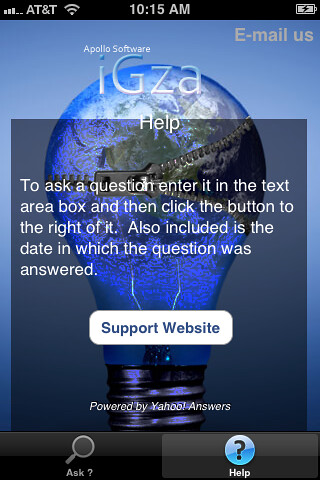The image is a screenshot of an earlier model iPhone displaying an app interface. At the top of the screen, the status bar shows three out of five white bars indicating signal strength, the AT&T carrier name, a Wi-Fi icon, and the time, 10:15 a.m. The battery appears nearly full. 

Within the app, the top right corner features an "email us" link, and below it, there's a logo reading "Apollo Software IGZA." Central to the screen is a help dialog overlay, which includes a black box with a light bulb and a zipper graphic. The text within this dialog instructs the user to "enter a question in the text area box and then click the button to the right of it." Additionally, it mentions that the date of the answered question is included, and users can access additional support via a white button labeled "support website," powered by Yahoo Answers.

At the bottom of the screen, there are two navigational tabs. The left tab, marked with a magnifying glass and the word "Ask?" in white text on a black background, and the right tab, showing a blue circle with a black question mark and the word "Help" in white text.